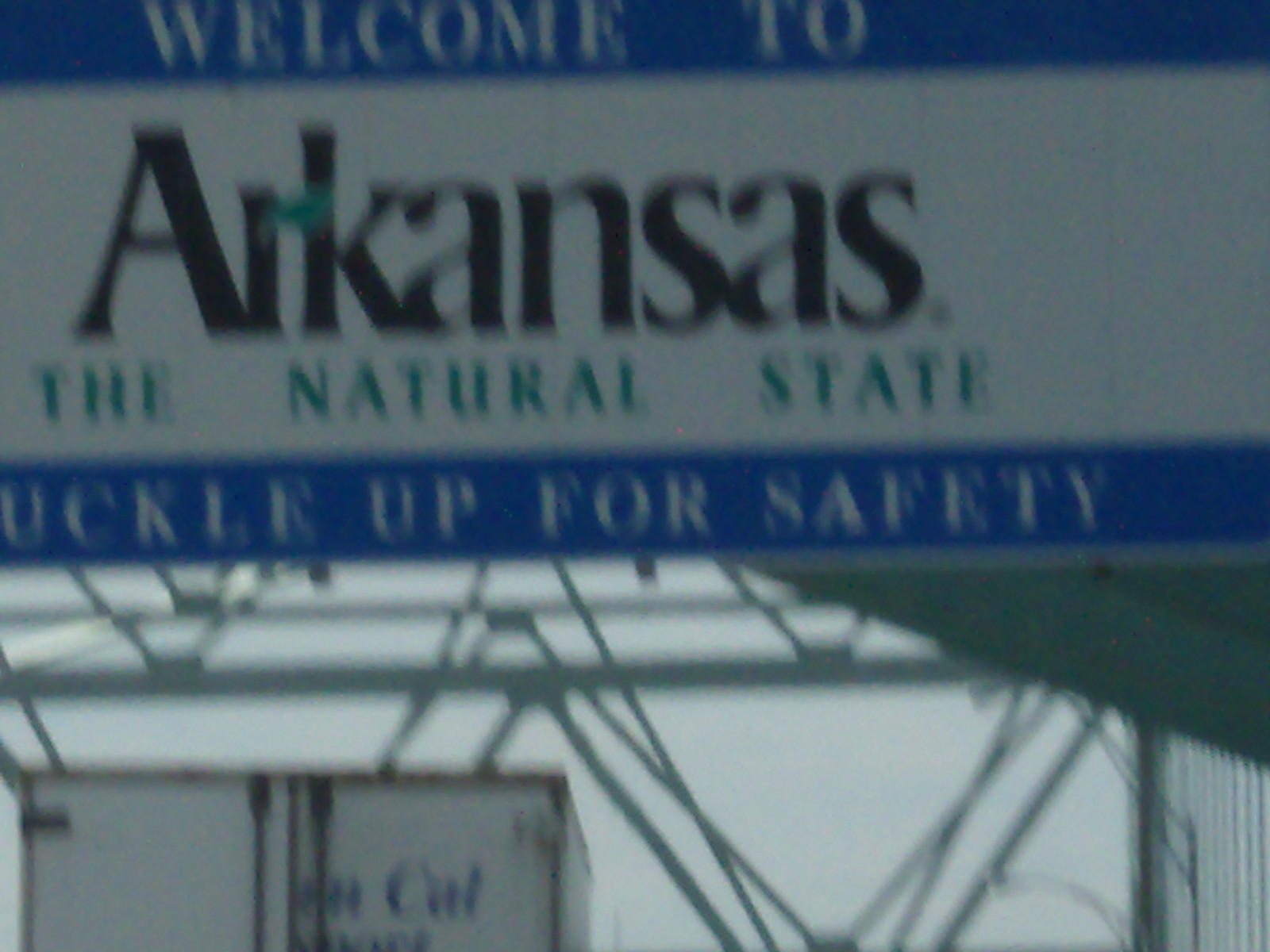The image depicts a rectangular, vertically oriented banner-type sign with prominent blue borders at the top and bottom. Within the top blue border, white lettering reads, "Welcome to Arkansas," while the middle section of the sign features text in a combination of green and black that states, "The Natural State." The bottom blue border also contains white lettering, partially cut off, displaying the message, "Buckle up for safety," with the first letter of the word "Buckle" obscured, leaving "Uckle up for safety." This sign is supported by a framework of steel rods, which are arranged to hold it firmly in place. The backdrop of the image is a gray, overcast sky, contributing to a somewhat somber atmosphere. Additionally, in the bottom left corner of the image, there appears to be a white box, likely the rear end of a truck, identifiable by its long, dark lines and hinge details along the edges.